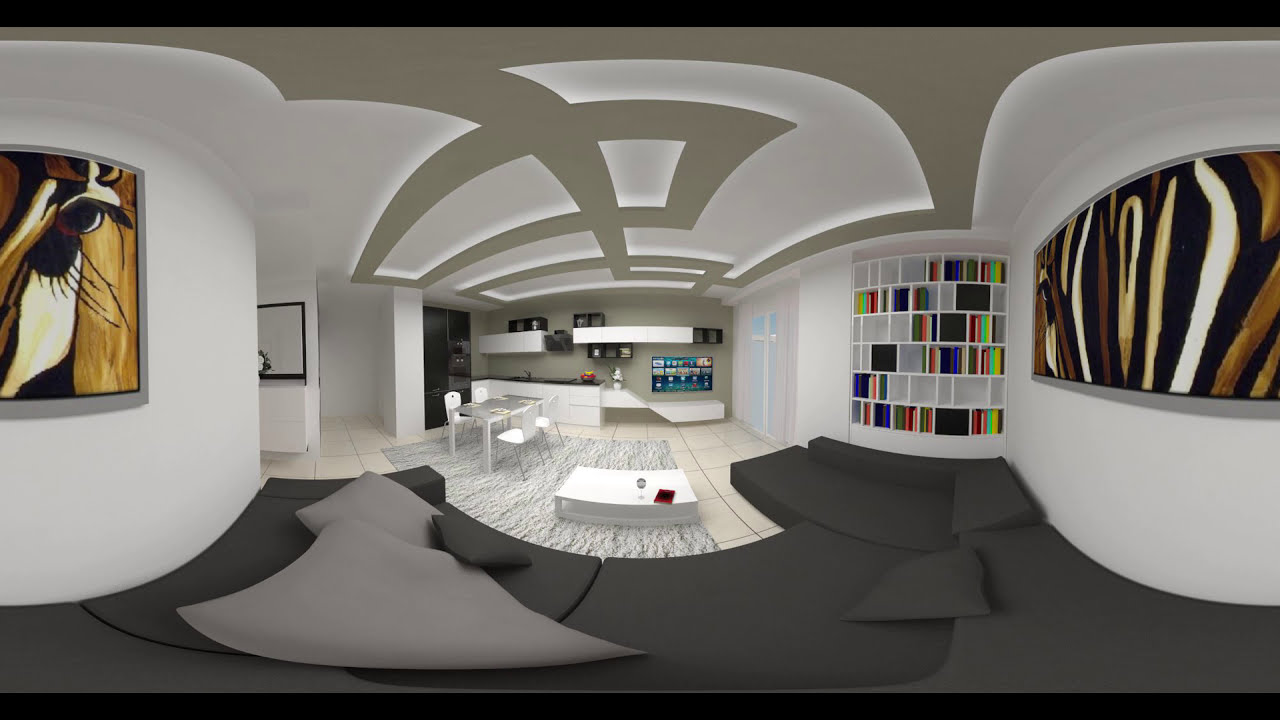This computerized mock-up presents an intricately designed living space with a distinctive, warped perspective that evokes a 360-degree or VR environment. The focal point is a dark gray, L-shaped sunken couch adorned with light gray pillows, situated around an inner area that features a light-colored rug atop a tiled floor. At the center of this setup is a low, white coffee table. 

To the right, there is an inset bookshelf filled with colorful book spines, adding a splash of vibrant hues to the room. On both the left and right sides of the image, the walls curve and feature abstract jungle safari-themed art. The left wall showcases an artwork that evokes the patterns of cheetah stripes, while the right wall displays a similar theme with animal-inspired patterns in browns, whites, and blacks. 

Against the far wall, white shelves and cabinets contribute a sleek, modern touch. Additionally, there is a tidy four-seater white dining set and a small glass table with white chairs positioned near it. The ceiling is adorned with a geometric cutout pattern, completing the contemporary aesthetic of the room. This image, intentionally devoid of any people, showcases a meticulously arranged indoor living space where the placement and flow of objects are balanced yet sophisticatedly scattered.